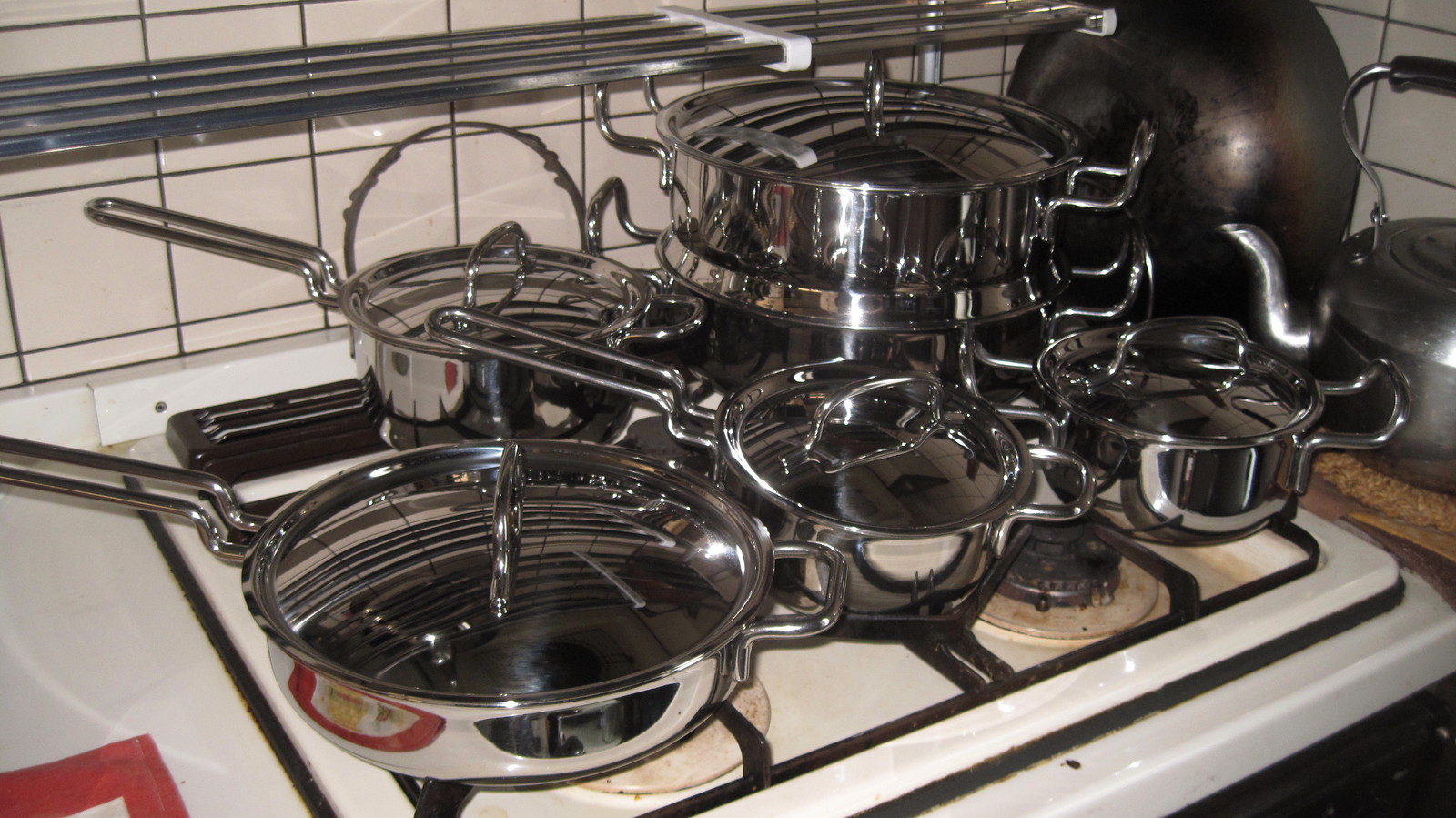This color photograph, taken inside a kitchen, captures a slightly dirty, white enamel gas stove with a black metal grate. The stove is laden with a brand new set of stainless steel pots and pans, all equipped with glass lids. Among the assortment are various saucepans, skillets, a large frying pan, stock pots, and notably, a double boiler. Each pot features wire-like handles, and the glass lids sport metal handles. To the right of the stove, on a brown countertop, rests a dull silver tea kettle and an upside-down stir-fry pan in silver and gray, leaning against the white tiled wall in the background. The tiles are square with black grouting, and a silver rack is mounted just above the stove, rounding out the kitchen setting.